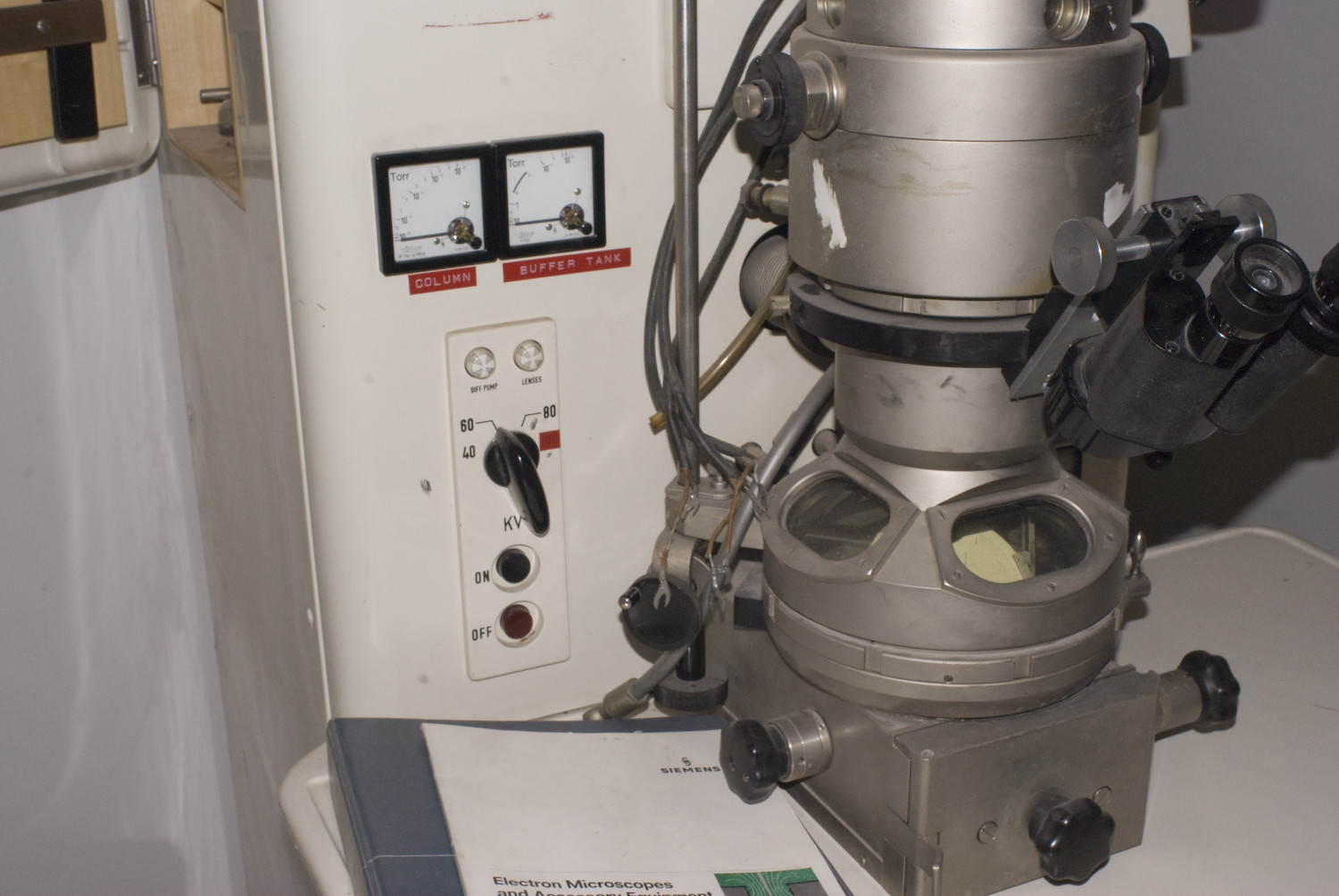The photograph, a rectangular image approximately 4 inches tall by 6 inches wide, depicts a detailed indoor scene centered around a scientific setup. Dominating the foreground is a light gray, almost plastic-textured table that starts from the lower right-hand corner, slopes slightly upward and then declines towards the left, not quite reaching the corner. On the left side of the table, there is a blue binder notebook with a smaller white pamphlet placed on top. The pamphlet features the Siemens logo in black print at the upper right-hand corner, with the visible text reading "Siemens" and "electron microscopes", though part of the title is cut off.

Adjacent to the pamphlet, a sophisticated, metallic scientific device is prominently displayed. This machine resembles a high-end microscope but is distinct from typical classroom models. It includes a large metal housing with a viewfinder, suggesting it's a specialized microscope. The device has an enclosure area, likely to contain samples securely. Black plastic knobs are situated around its base.

Mounted on the white wall behind the device is a panel featuring two square gauges, each outlined in black. The left gauge has a red bar and white print reading "column," while the right gauge, also red with white print, reads "buffer tank." Below the gauges is a vertical panel containing further controls. At the top are two knobs, where the left is labeled "DIFF pump" and the right "lenses." Below these, there's a black turn knob marked with increments starting at 40, currently set at 60, and maxing at 80 on the right. The bottom part of this vertical panel has the notation "KV," and beneath it are two buttons: a black one labeled "on" and a reddish-brown one marked "off."

The detailed layout, scientific instrumentation, and variety of controls depicted attest to a professional lab setting, emphasizing precision and complexity in the equipment shown.